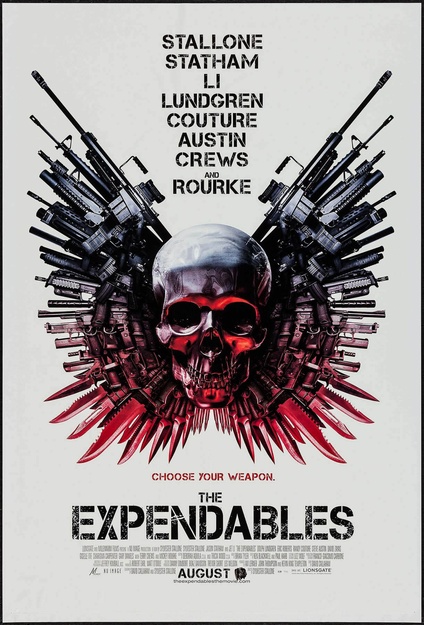A promotional movie poster with a light gray background and bold black text prominently lists the names of the cast: Stallone, Statham, Lee, Lundgren, Couture, Austin, Cruz, and Rourke. Dominating the center of the poster is a striking image of a skeleton head, colored in shades of gray and red. The skull, adorned with large, menacing teeth, is surrounded by an array of silver and black guns extending outward from its head in a formation reminiscent of butterfly wings. Complementing this arsenal, intricately positioned red knives fan out from the bottom, adding to the poster's intense and dark aesthetic. A bold caption at the bottom reads, "Choose Your Weapon," followed by the title, "The Expendables." This vividly detailed poster captures the intense and thrilling essence of the forthcoming movie, evoking a sense of suspense and danger.